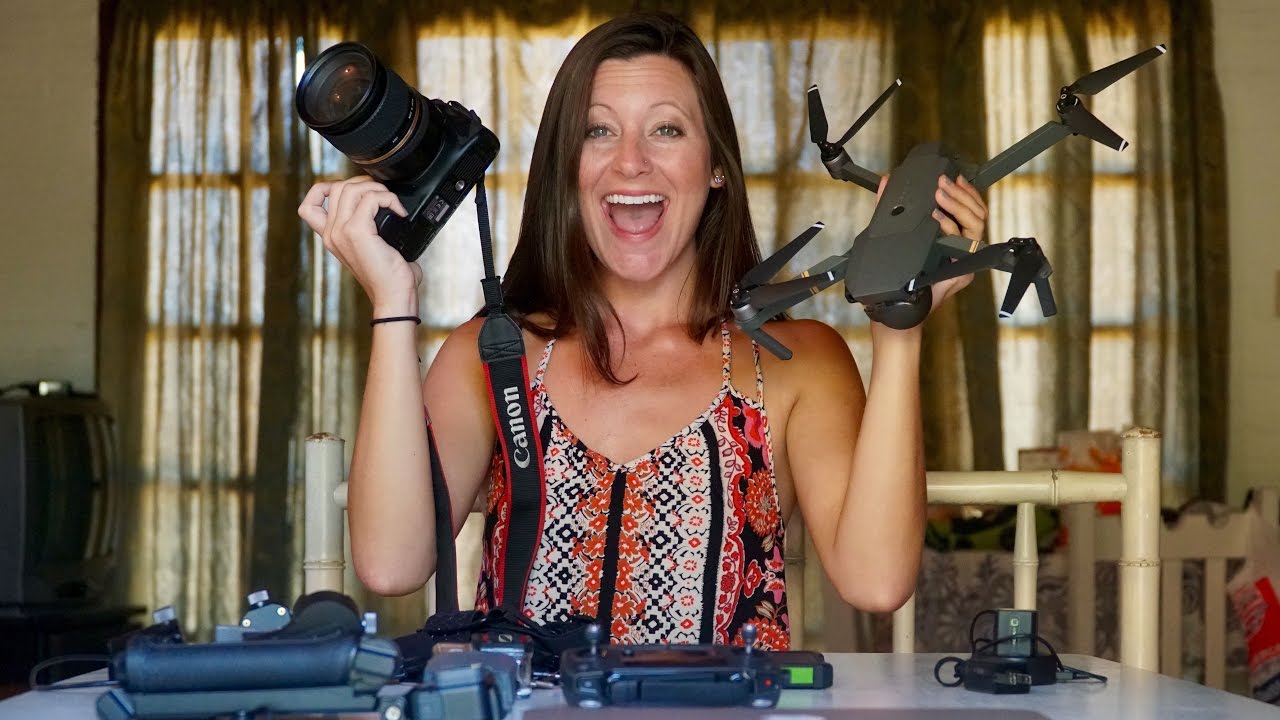In this vibrant image, a woman with long brown hair is captured from the torso up, smiling widely with her mouth slightly open, exuding a feeling of surprise and happiness. She holds a gray drone with four propellers in her left hand and a camera, which has a lens and a Canon-branded strap, in her right hand. The woman is dressed in a spaghetti strap tank top featuring an intricate pattern of red, orange, white, and black designs. She stands in what appears to be a living room, with a large window behind her draped in brown transparent curtains, allowing sunlight to filter through. In front of her is a counter or table cluttered with various electronic accessories, including a black drone remote controller and a black camera carrying case. The room features off-white beige walls, and to the left of her, there is a TV in the corner, while to the right, there’s additional furniture and boxes. The table in front of her is gray and loaded with various pieces of camera equipment.